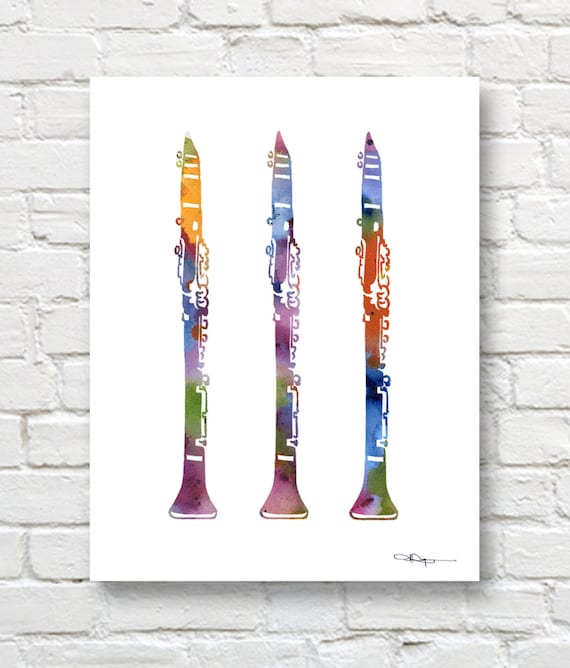This image is an art piece featuring an illustration of three stylized, multicolored clarinets (mistakenly referred to as flutes and soprano saxophones). They are meticulously aligned vertically, side-by-side, each presenting a vibrant gradient of colors that blend seamlessly, likely created with watercolor paint. The first clarinet on the right starts with an orange mouthpiece and transitions through blue, green, and purple. The second clarinet begins with a blue mouthpiece, adorned with white stripes, and flows through shades of purple, green, blue, and light purple. The third clarinet has a blue mouthpiece as well, with its body transitioning from green to red, blues, and finally merging with green and purple at the bottom. The piece is signed by the artist in the lower right corner, though the signature is difficult to decipher, possibly reading "GAP." The illustration is set against a white background and is mounted on a white painted brick wall, adding to its striking visual appeal.